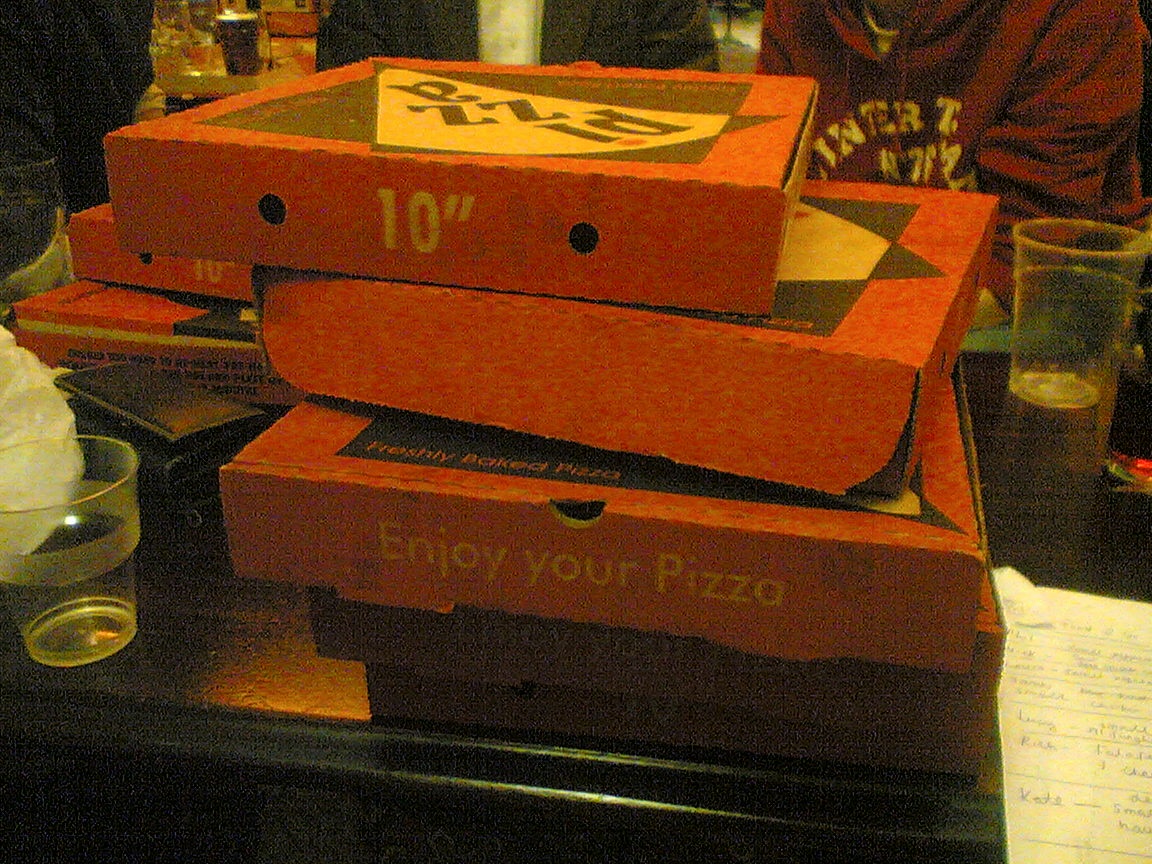In this slightly blurry, dimly lit photograph, a cluttered scene on a dark wooden table or countertop comes into focus. Dominating the front center are four square, red pizza boxes stacked on top of each other. The top box displays a black square logo with a white triangular pizza slice that reads "PIZZA" in bold black lettering. The text "10 inch" is printed on the side of this box, and two holes are cut out of its cardboard. The second box from the bottom features the words "enjoy your pizza," and below it, another box reads "freshly baked pizza." 

To the left of the front stack, a short empty glass stands, while to the right a white rectangular receipt is visible. In the background, additional pizza boxes are stacked haphazardly, reinforcing the impression of a recent pizza party or gathering. Seated behind the main stack, two people are partially visible; one wears a red sweatshirt with white writing. The overall ambient setting suggests a cozy indoor environment, possibly a restaurant or a casual gathering space.